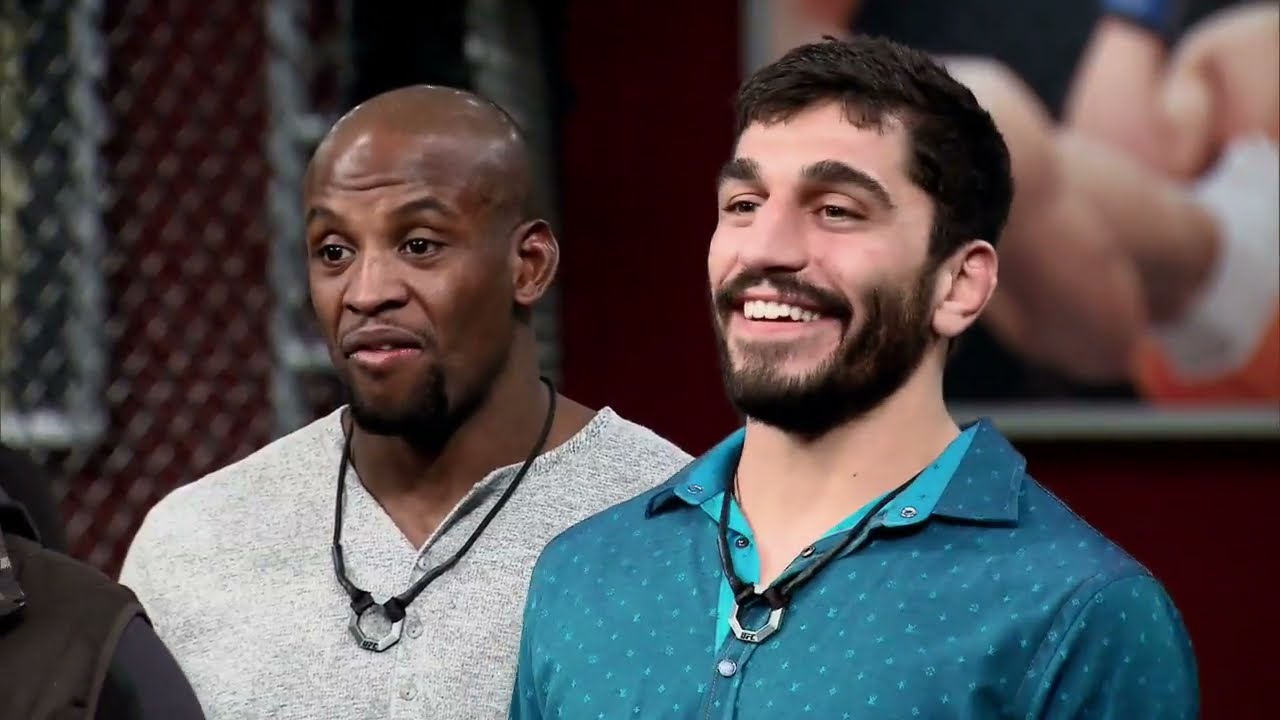The photograph captures two men standing side by side, looking off to the left, seemingly engaged in a conversation or listening intently to someone. The man on the left is black, bald, and is donned in a gray heather Henley shirt. He has facial hair on his chin and above his lip, and he's wearing an octagonal silver pendant on a black cord around his neck. The man on the right is Caucasian, with short black hair, prominent eyebrows, and brown eyes. He sports a deep green sports shirt with snap-up buttons and has a well-groomed short black beard. He is smiling broadly, revealing very straight, white teeth. He, too, is wearing an identical octagonal silver pendant on a black cord. The backdrop suggests a professional sports setting, possibly a locker room or an athletic club, given the blurred artwork depicting figures in gloves and trunks, indicative of boxing or martial arts. Additionally, there appears to be an LCD screen behind the Caucasian man, displaying a crowd scene.